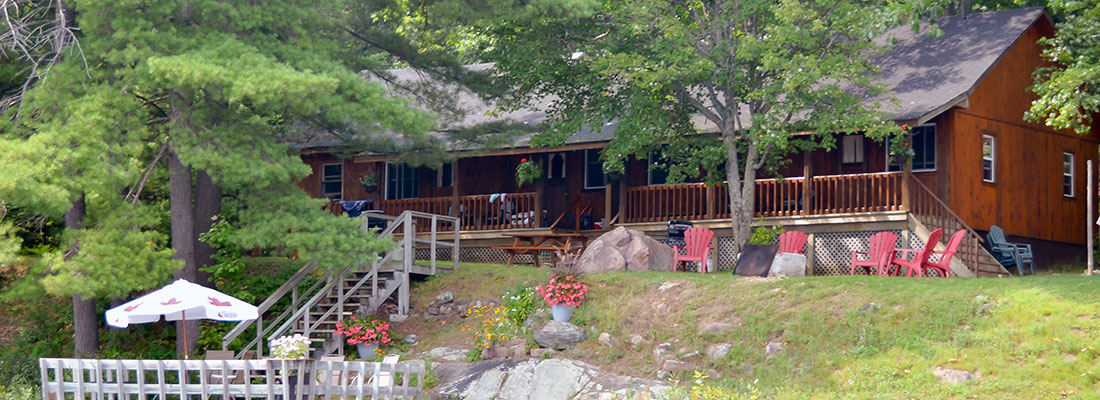The photograph depicts a picturesque, expansive wooden farm-style house resembling a large log cabin, characterized by its rich, dark brown wood and numerous windows that adorn the front. The house features a substantial wooden porch with a matching railing, beneath which are five bubblegum pink chairs scattered about. A hanging potted plant is suspended from the porch ceiling. The house has a sloping, grayish roof and is surrounded by tall green trees.

The foreground showcases a slight, grassy hill dotted with rocks and decorated with white pots that bloom with pink and white flowers. In the lower left-hand corner, a charming white picket fence encloses a patio area, where a white umbrella with pink or red patterns provides shade. Wooden stairs lead down from the porch to this patio area, hinting at the presence of water nearby as the grass slopes into rocks, suggesting a river just out of sight. This serene backyard scene is complemented by additional wooden furniture, including a wooden chair leaning against the house and another wooden enclosure under the umbrella, adding to the cozy and inviting atmosphere.